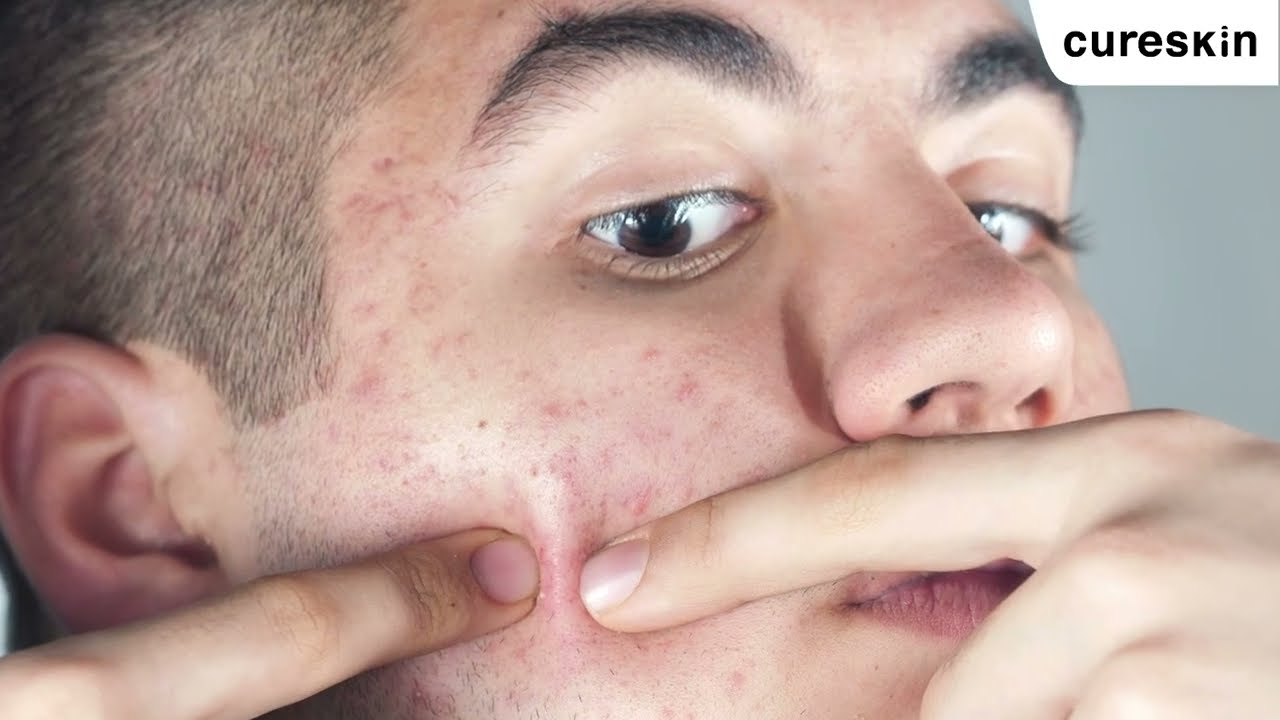The image is a detailed advertisement for the company Cure Skin, featuring their logo in the top right corner. The logo is in all black, lowercase letters on a white background, with a distinct half-moon shape over the "i" in "skin." The rest of the background is gray, highlighting a close-up of a young man with significant acne. He has very short hair, almost shaved, with a bit of hair visible. His bushy eyebrows and brown eyes are focused intently on his fingers, which are poised on his face as if ready to pop a pimple. Both his index fingers touch his cheek, and his fingernails are neatly trimmed. The lighting is good, suggesting an indoor setting, and the entire bottom portion of the image is dominated by the man's face and hands. This ad clearly aims to promote a product designed to address acne issues.